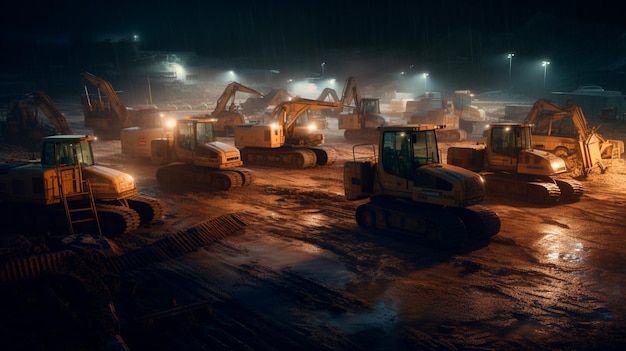The image depicts a dark, nighttime scene of an outdoor construction site that appears to have recently experienced rain, as indicated by the wet, muddy ground and several visible puddles. Dominating the scene are numerous pieces of yellow construction equipment, including bulldozers, diggers, and possibly cherry pickers, arranged throughout the yard. There are at least five machines prominently visible, with more in the background. A network of floodlights and streetlights illuminates the area, casting reflections on the wet ground and providing much-needed light. In the distance, one can make out faint outlines of trees and a glimpse of the moon, suggesting the setting is outdoors under a dark night sky.